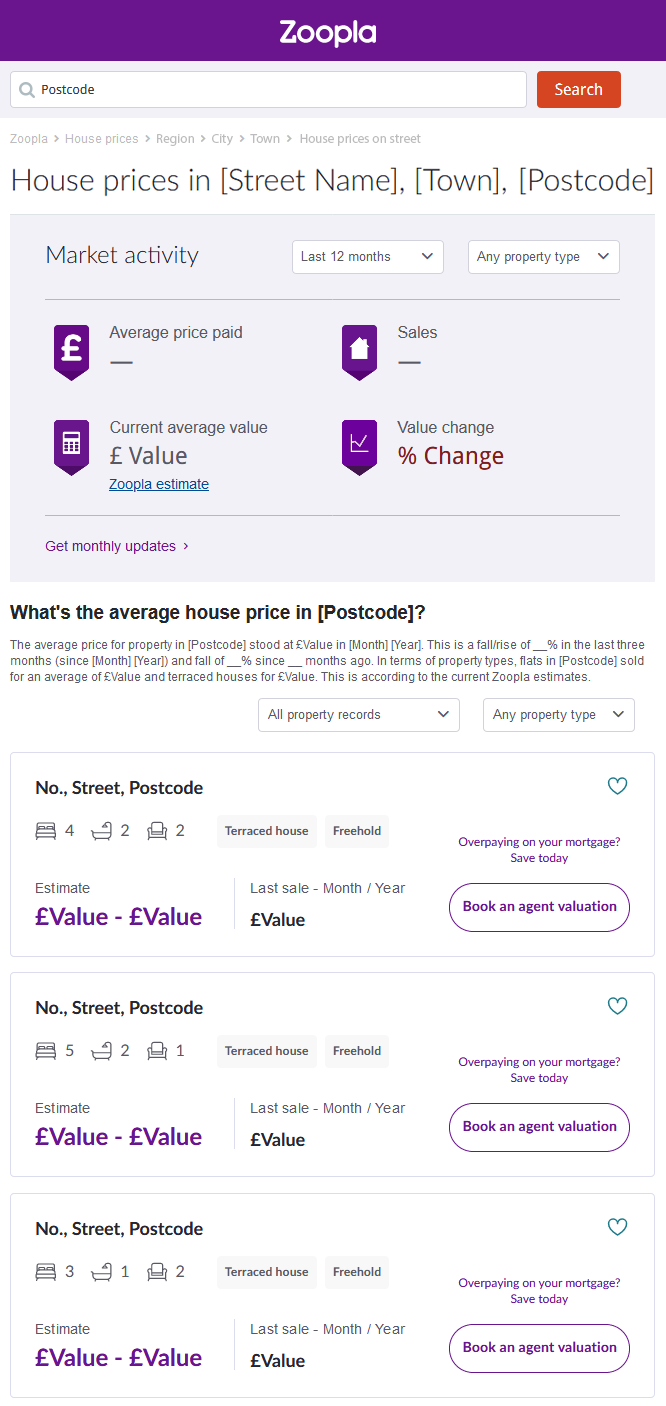This is an image of the Zoopla website interface. The Zoopla logo, written in white text, is prominently displayed on a purple background, creating a striking visual contrast. In the center-right of the image, there is a white section featuring various search functionalities. 

A search bar labeled "postcode" is accompanied by a small magnifying glass icon, and situated next to it is a red button that says "search." Beneath this, there are menu options for navigating Zoopla's features, including sections for house prices by region, city, town, and street. This also includes specific filters showing details like the house prices on streets with their town and postcode in parentheses.

The page displays market activities over the last 12 months for any property type, with details including the average price paid, number of sales, current value, value change, and percentage change. Users can opt for monthly updates and find the average house price within a specified postcode. 

Property listings on the site provide extensive details such as the value, number of bedrooms, and number of baths, visually represented by icons for beds, baths, and chairs. 

On the right-hand side, there's an option to book an agent valuation, highlighted in purple text and numbers. Additionally, users can mark properties as favorites by clicking on heart icons next to the listings. Most of the text on the page is in black, while key elements like "value" and "booking the agent" are color-coded in purple for emphasis.